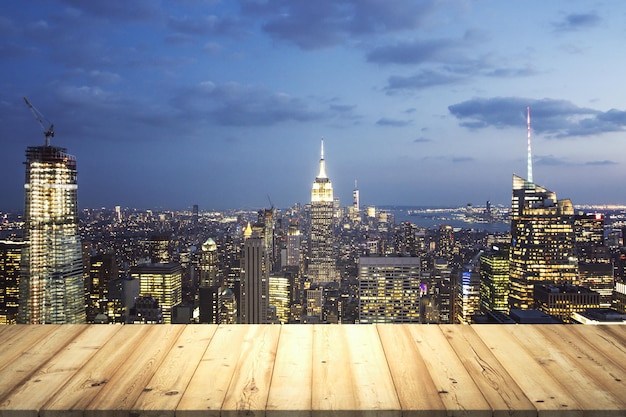Captured from a high vantage point within a towering building, this image offers a sweeping view of a sprawling city skyline, most likely New York City. The iconic silhouette of the Empire State Building rises prominently among the skyscrapers that stretch across the horizon. The vantage point is so elevated that several of the surrounding structures appear level with the photographer's perspective. The sky, painted in gentle hues of sky blue, hints at the approaching sunset, casting a serene glow over the urban landscape.